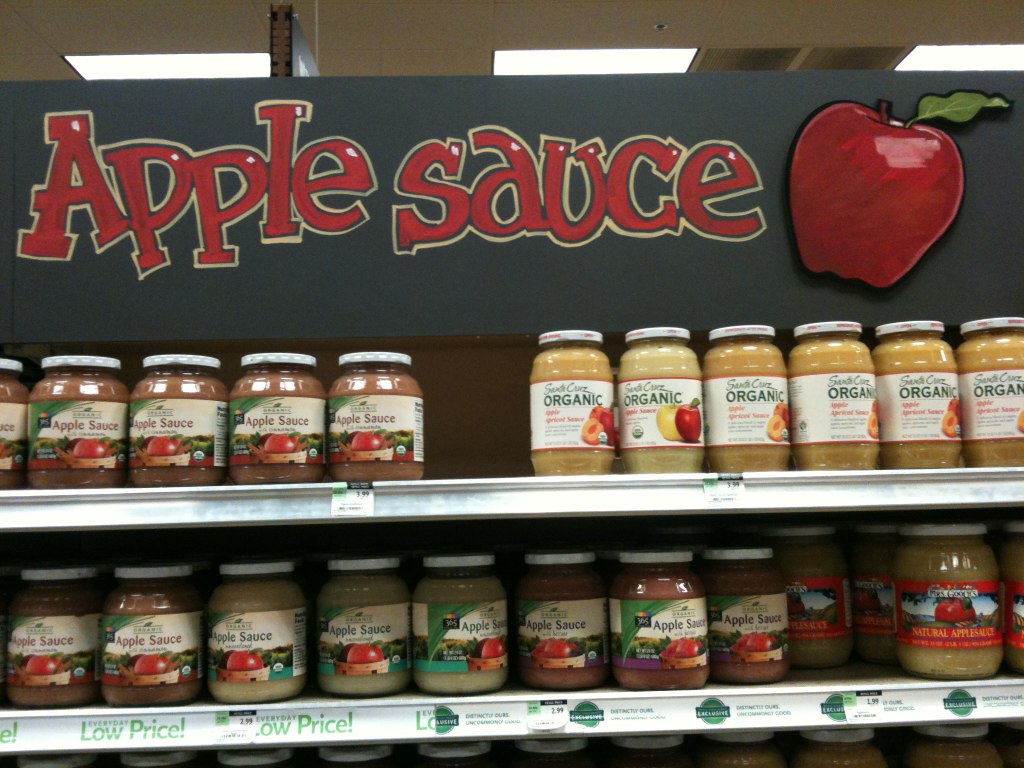In the image, you see a close-up of a neatly organized grocery store aisle, likely an organic grocery store given its upscale appearance. Prominently displayed at the top of the shelves is a large black rectangular sign with bold red letters spelling out "applesauce," bordered in white. Adjacent to the text is a drawing of a shiny red apple complete with a brown stem and a green leaf. Below this sign, the top shelf showcases various jars of applesauce. The jars on the left are shorter and thicker, filled with a darker, almost brown-red applesauce, and labeled with "applesauce." Their price tags read $3.99. To the right, there are taller, skinnier jars containing lighter tan-apricot colored applesauce with labels indicating it's organic. These jars are priced the same at $3.99.

The second shelf continues the display with a range of jars varying in size and color, from classic light tan to deeper, more purplish hues. Price tags range from $1.99 to $2.99. This shelf includes repeated "everyday low price" stickers, and each jar consistently has a white lid. The third row is mostly cut off in the image, but you can see the tops of more jars, indicating a continuation of the applesauce display. Additional stickers on the shelves display varied prices, though not all are clearly visible. The assortment of jar sizes and applesauce colors, along with the detailed labeling, highlights the store's diverse selection of applesauce offerings.